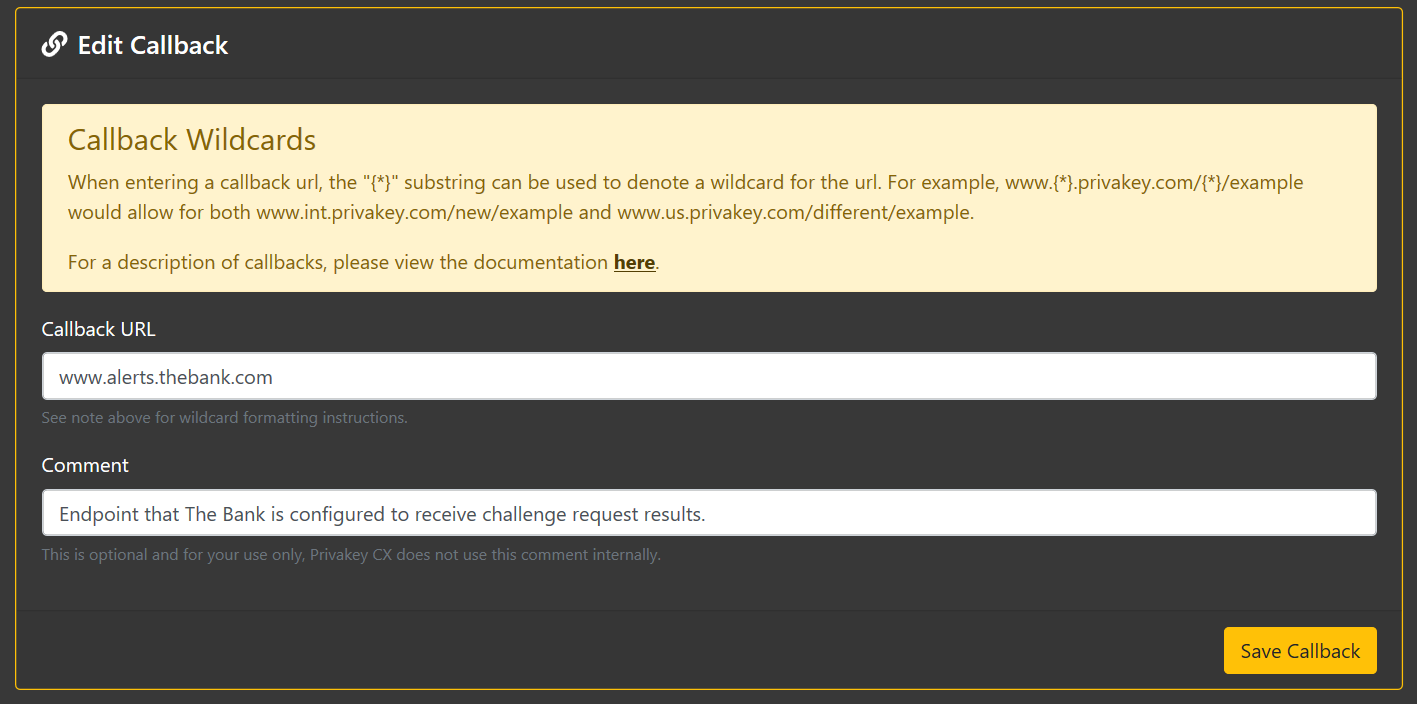In the image, the background is entirely black with various elements arranged predominantly towards the top left and bottom right corners. 

1. In the top left corner, there is white text that reads "Edit Callback" accompanied by a link icon to its left.
2. Directly below this, there is a light yellow rectangle with the text "Callback Wildcards" written in a larger font. Beneath this heading, in smaller font, there is a detailed instruction:
   - "When entering a callback URL, the (*) substring can be used to denote a wildcard for the URL. For example, www.*privatekey.com would allow for both www.intprivatekey.com/new/example and www.usprivatekey.com/different/examples. For description of callbacks, please use documentation here." The word "here" is bold and underlined.
3. Below the yellow rectangle, there is a white input box labeled "Callback URL" which displays the URL "www.alerts.thebank.com."
4. Further down, there is another label "Comment" in white text, under which it says "End point that the bank is configured to receive challenge request results."
5. In the bottom right corner of the image, there is a gold rectangle with the text "Save Callback" written in black.

This detailed caption clarifies the contents and structure of the interface depicted in the image.